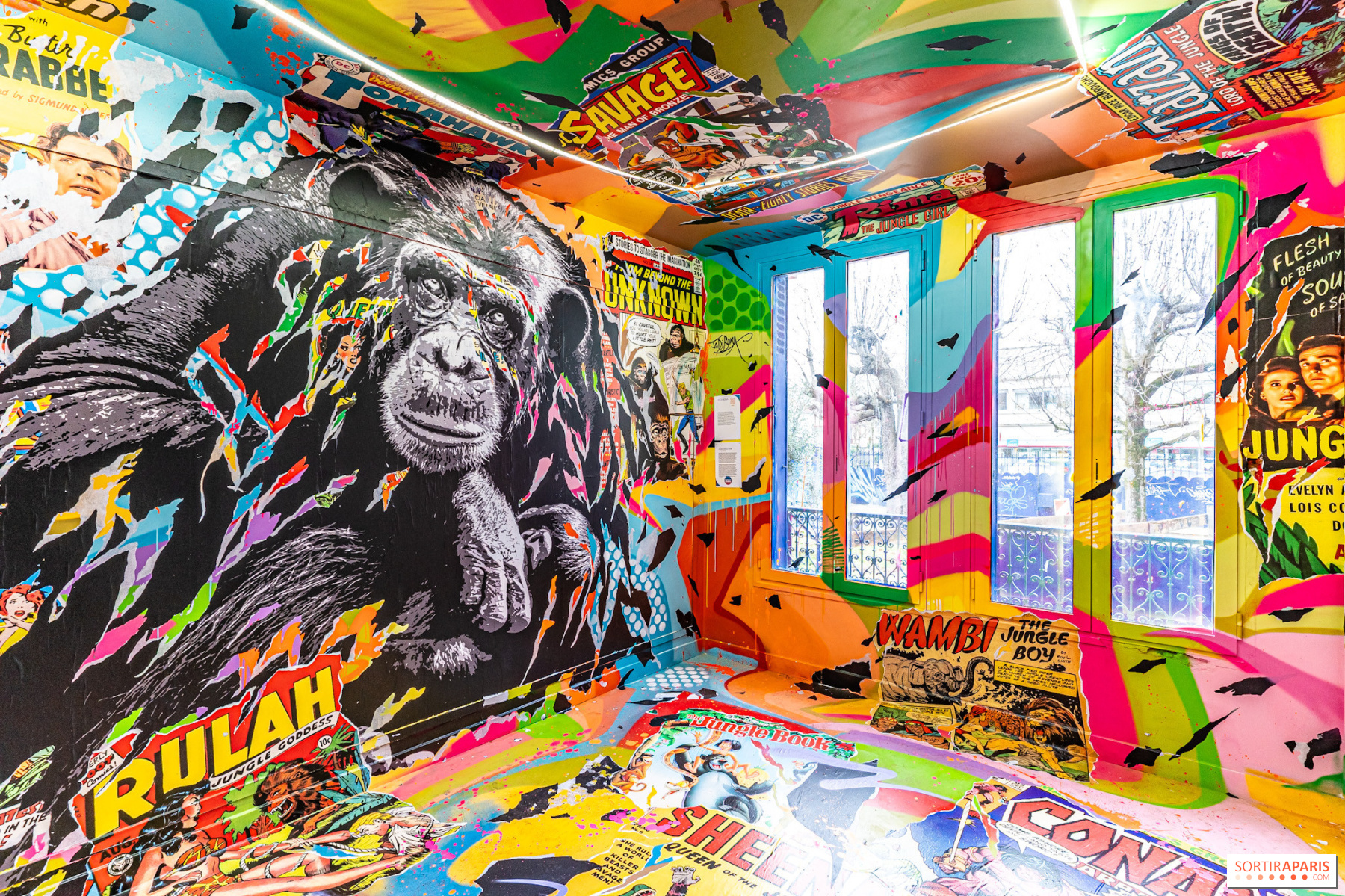The photograph captures a vividly colorful and lively interior room, rendered in a graffiti and comic style that envelops the floor, walls, and ceiling. On the left wall, a large, imposing black-and-white depiction of a chimpanzee, with its arms bent under its chin, draws immediate attention. The mural extends from the floor to the ceiling and is accented with splashes of bright, fluorescent colors. Below the chimpanzee, bold yellow letters spell out "R U L A H" against a red background. On the right wall, a series of four rectangular windows allows natural sunlight to flood the space, illuminating the dense array of stenciled, drawn, and painted movie posters and cartoon-like images that cover every visible surface. The entire room is a riot of colors, including vibrant shades of yellow, orange, blue, red, pink, purple, and green, forming an eclectic, collage-like display without any furniture to interrupt the visual feast. The windows reveal a glimpse of a courtyard or yard, adding to the dynamic and busy atmosphere of this uniquely decorated room.